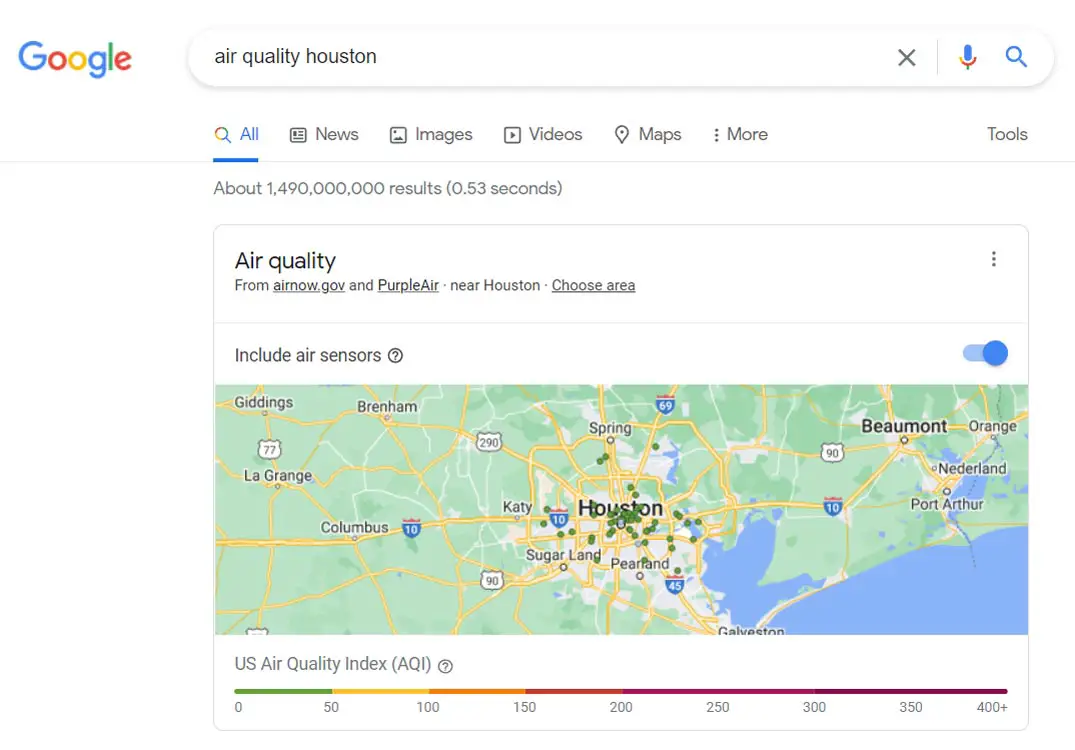**Detailed Caption:**

This image is a cropped screenshot of a Google search results page. At the top left corner, the Google logo is prominently displayed. To the right of the logo is the search bar, where the query "air quality houston" has been entered in all lowercase letters. 

Beneath the search bar is a horizontal navigation menu with several options: "All," "News," "Images," "Videos," "Maps," and "More." Currently, the "All" tab is selected and highlighted in blue with a corresponding blue underline indicating active status.

Below the navigation menu, the search results summary indicates approximately 1.49 million results found in 0.53 seconds.

The main section below the summary features a dedicated information box. At the top left of this box, a heading reads "Air quality." Immediately below, there's a source attribution from "airnow.gov" and "PurpleAir" with a location note for "near Houston." An interactive link labeled "Choose area" is underlined, suggesting functionality to select a different geographic area.

To the left within this box, there's an option labeled "Include air sensors," adjacent to an active toggle switch set to the "on" position.

Occupying the lower part of this information box is a detailed map of Houston, studded with green and blue dots indicating various air quality monitoring points across the city. Beneath the map, the label "US Air Quality Index" is accompanied by a color-coded line graph that correlates with the colored dots on the map, providing a visual representation of the air quality data.

This comprehensive search result layout serves as a powerful tool for quickly assessing current air quality conditions in Houston through both textual information and interactive visual elements.